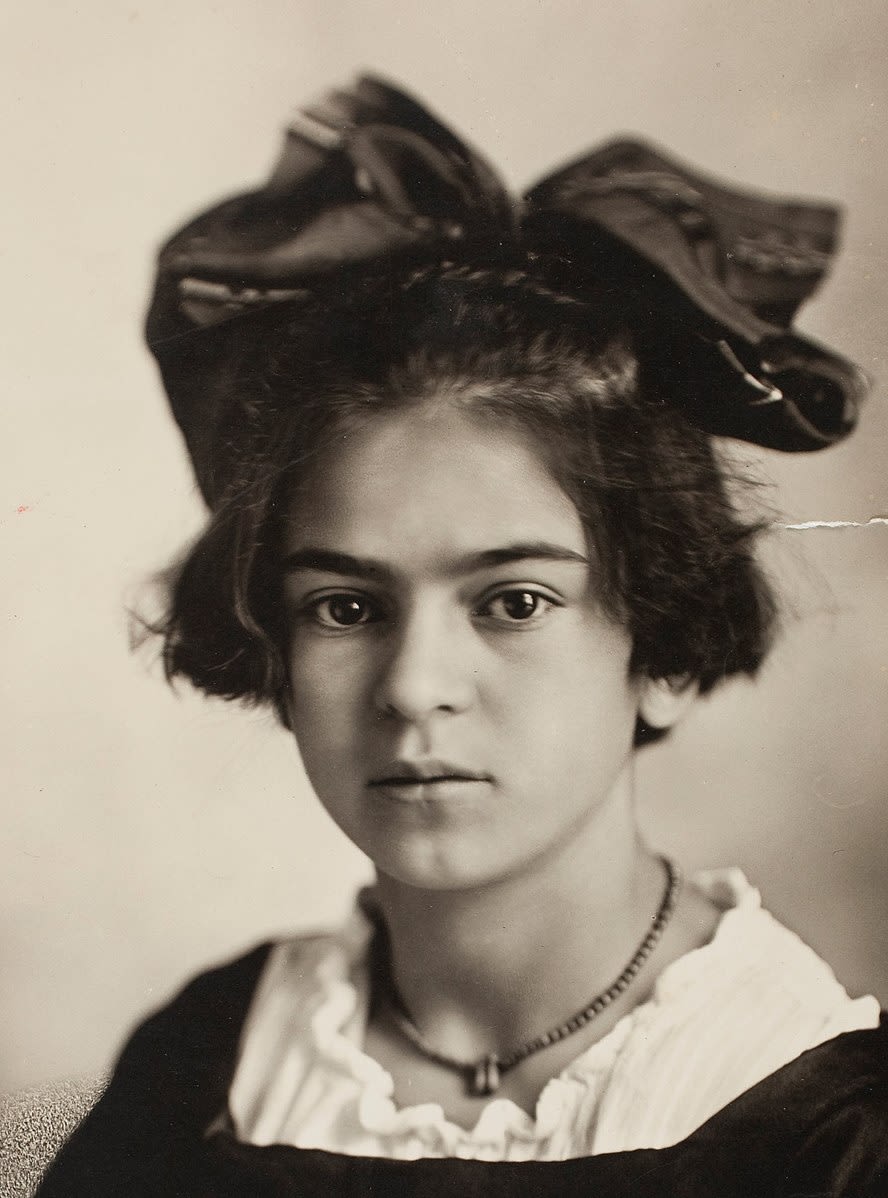This is a detailed black and white photograph, likely from the 1940s, capturing a young woman from the shoulders up. She has dark, ear-length hair that is straight but slightly frizzy, with matching dark, natural-looking eyebrows and dark eyes. Perched on the back of her head is an elaborate bow or hat. Her fair skin contrasts with the serious expression on her face as she gazes intently into the camera. The woman wears a dark dress featuring a white lace collar, over which she dons a necklace that aligns with the neckline of the blouse. The overall look, including her plain yet classic attire and jewelry, suggests an older style reminiscent of the era. The background is plain, enhancing the vintage feel of the image.